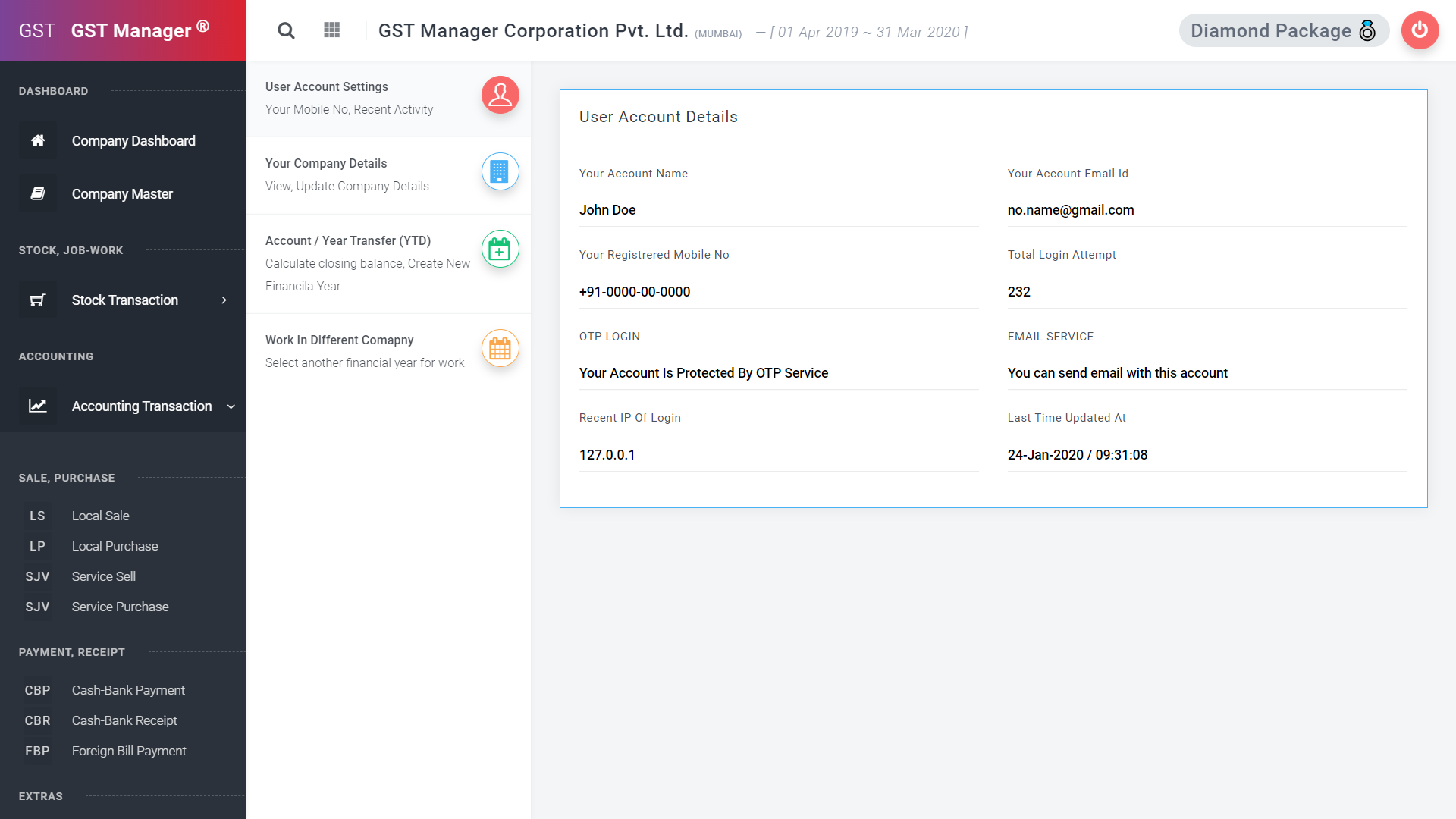The image depicts a user interface of a web-based application with a predominantly white, gray, and dark blue or black color scheme accented by colorful icons. At the top of the interface, there's a navigation bar labeled "GST Manager Corporation, PVT, LTD," followed by a date range spanning from April 2019 to March 31, 2020. On the right side of this bar, it indicates the "Diamond Package," accompanied by a small red power button icon. The far left of this bar reiterates the application's name, "GST Manager."

Below this top bar, a sidebar pane colored in black displays a series of clickable sections in white text. These sections include options such as Dashboard, Company Dashboard, Company Master, Stock Transaction, Accounting Transaction, Sale Purchase, Local Sale, Local Purchase, Service Self, Service Purchase, Payment Receipt, Cash Bank Payment, Cash Bank Receipt, and Foreign Bill Payment.

The main interface, primarily white and gray, is dedicated to user account settings. In this section, you find fields for entering user and company details. Sample placeholder details are provided: the account name is listed as John Doe, the mobile number as 919-000-000, and the account is protected by OTP service. The recent login IP is shown as 127.00.0, and the account email is displayed as noname@gmail.com. These placeholders indicate the sections where actual user information can be inputted.